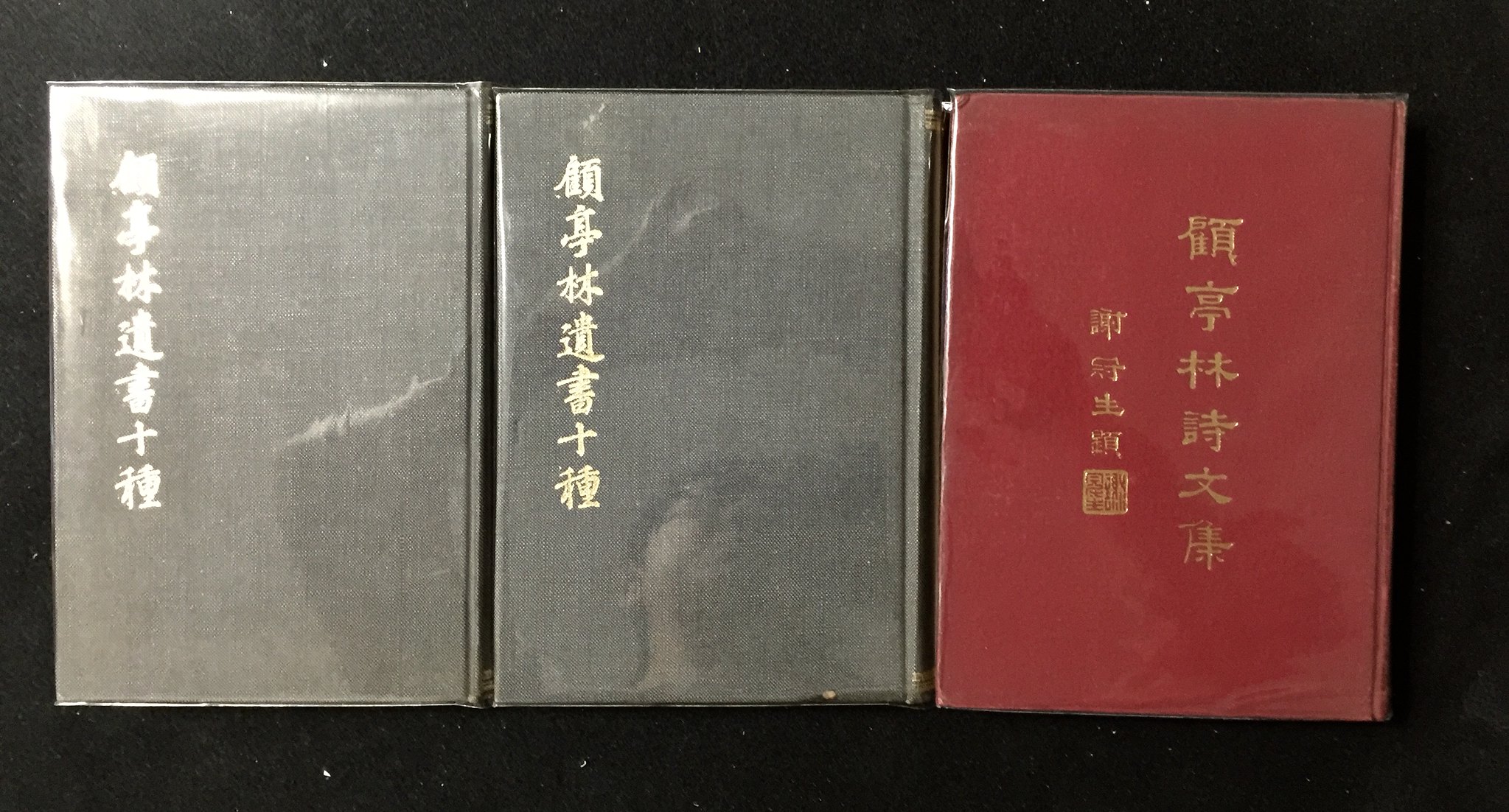This color photograph captures three seemingly old leather-bound notebooks lying on a black surface, which is speckled with a few white spots likely caused by light reflections. A light source from the left illuminates the scene, causing glare on the upper left-hand corner and just right of the center of the first notebook. The two notebooks on the left are gray and feature vertical lines of Chinese characters, printed about halfway down the left edge. The characters on the leftmost notebook are white and somewhat blurry, mirroring the clearer goldish-white characters on the second gray notebook. The rightmost notebook, in contrast, has a maroon or rust-colored cover with two vertical columns of different Chinese characters, positioned one-third of the way in from the left edge. These characters do not match those on the gray notebooks and are arranged with six symbols in the left column and five in the right. The shiny covering on the gray notebooks reflects the light, adding a glisten to their worn surfaces.